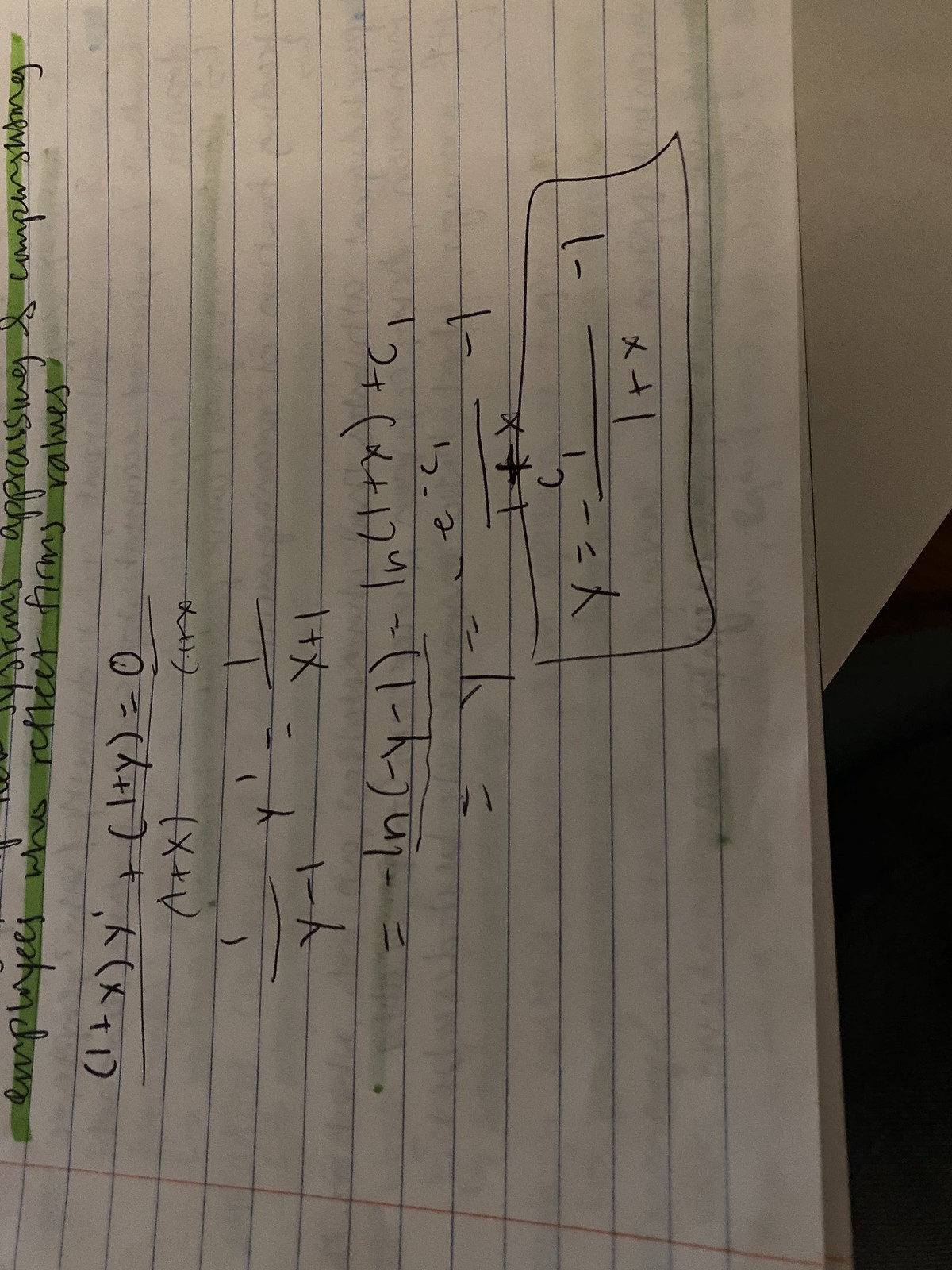Here's a cleaned-up and detailed descriptive caption for the image:

---

An indoor color photograph captures a notebook page on a countertop or desktop. The image, despite being dark, is in sharp focus. The notebook page is oriented 90 degrees to the left, making the handwritten notes appear vertically. The page contains an equation that someone is attempting to solve, written in pen. 

Starting from the top, the equation reads: 

\[
(1 + X)(Y^1) + (1 + Y) = 0
\]

Below this, in a new line, it continues with:

\[
\frac{1}{1 + X}
\]

Further down, the following expression is written:

\[
\frac{1}{Y} - Y \cdot Y^1 = \frac{1}{X + 1}
\]

The subsequent line states:

\[
= -1 - Y - Y = 1 + (1 + X) + C_1
\]

Next, the equation progresses to:

\[
Y = e^{-C_1} \frac{1}{1 + X} - 1
\]

Finally, in the lower right-hand corner of the image, enclosed in a rectangle, it reads:

\[
Y = \frac{C_1}{1 + X} - 1
\]

Additionally, along the left edge of the page, there is text highlighted in green, but despite the highlighting, this text is also written in pen.

---

This caption ensures a clear and detailed description of the image's content.